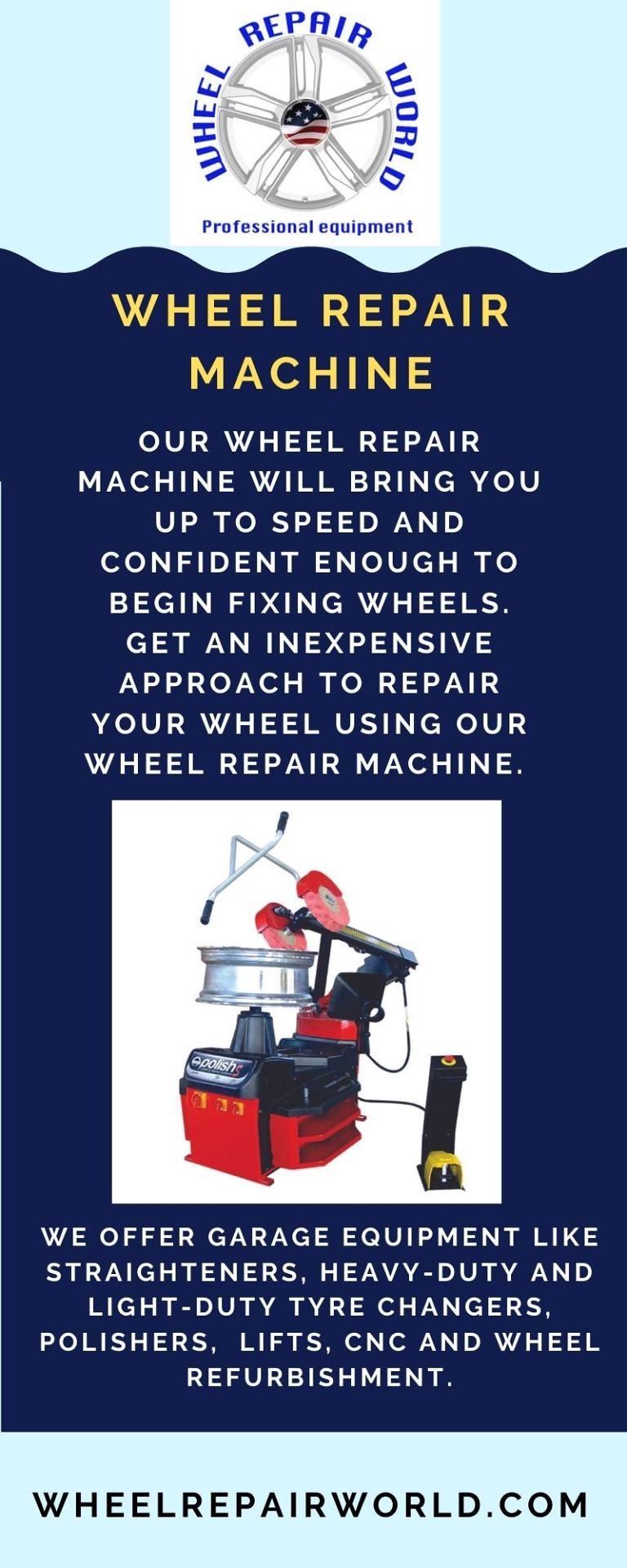This color advertisement for Wheel Repair World prominently showcases their Professional Equipment offerings. At the top, against a sky blue background with wave-like trim, the company’s logo features a silver wheel with blue font underneath reading "Professional Equipment." Below, on a dark blue background, bold yellow text announces the "Wheel Repair Machine." The advertisement emphasizes that this machine will make you confident enough to start fixing wheels, offering an inexpensive solution. A detailed list follows, highlighting available garage equipment such as straighteners, heavy-duty and light-duty tire changers, polishers, lifts, CNC machines, and wheel refurbishment tools. A notable feature is an image of the wheel repair machine, resembling a complex gadget or drum-like device, along with the website, www.wheelrepairworld.com.